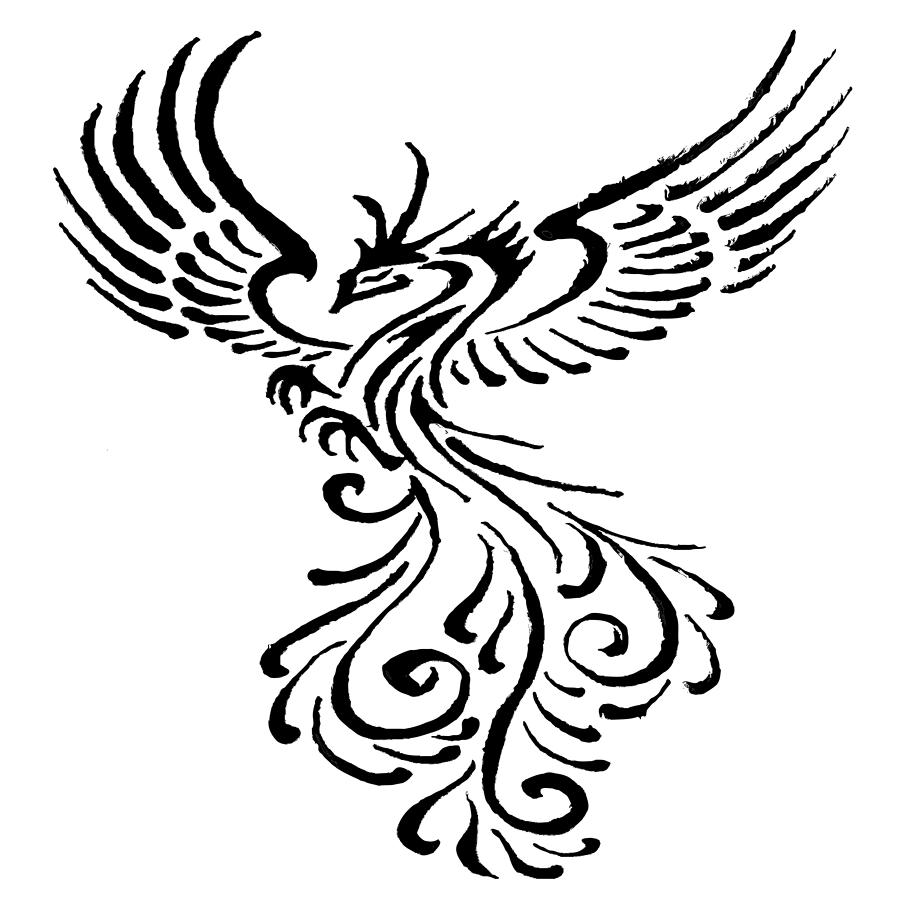This image is a black and white line art illustration of a fantasy bird, resembling a majestic phoenix with possible peacock influences. The bird is depicted with its wings spread wide, arching upwards on either side. Its head faces left, featuring a thick pointed beak, three long claw-like crests on top, and four sharp ridges down the back of its neck. The bird's body is adorned with several black streaks, while its claws, each with three sharp curved talons, extend outwards. The lower half of the image is dominated by the bird's extravagant tail, embellished with swirling black lines down the center and additional black curves around each edge. The entire scene is rendered with intricate black lines against a pure white background, showcasing ornate details and flowing designs throughout the bird's feathers.